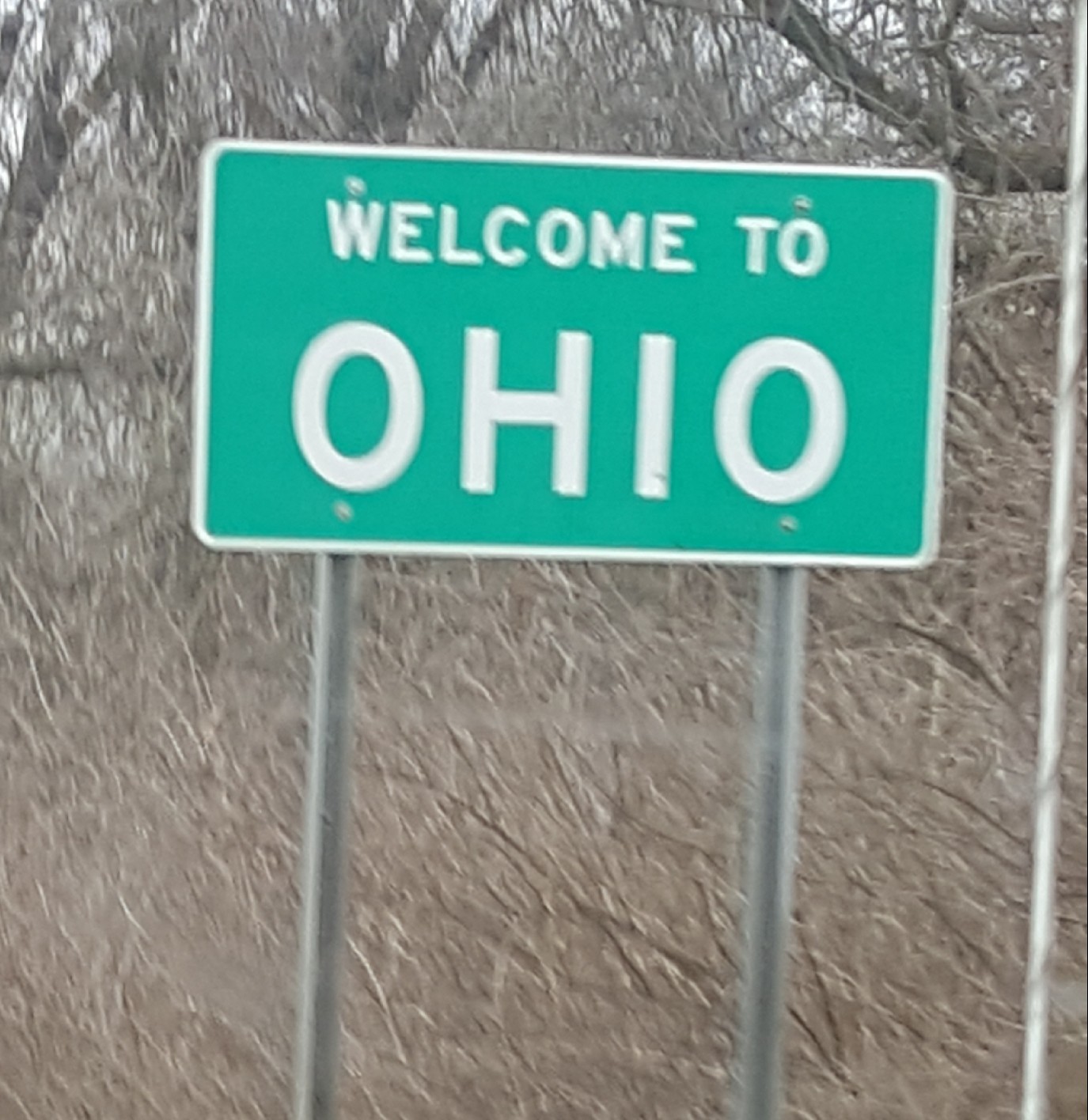A slightly blurry photograph taken outdoors of a tree-lined area. The background is filled with a tangle of bare branches, suggesting the season is winter due to the absence of leaves. The picture, possibly taken from a moving car, displays a slight motion blur. Prominently in the foreground stands a highway sign. It is fixed onto two gray poles and features a green, rounded rectangular board outlined in white. The sign reads "WELCOME TO OHIO" in uppercase white letters, with visible bolt details securing the sign to its poles.